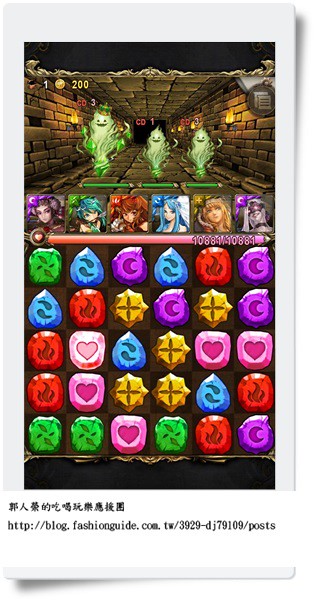The image is a detailed screenshot of a cell phone app that appears to be a puzzle game similar to Candy Crush. The bottom of the picture features Chinese characters and a web address, blog.fashionguide.com, which suggests it might be a promotional or hosted game. The main gameplay area consists of a grid with five rows of various colored and shaped jewels adorned with different symbols such as hearts, flames, crosses, and leaves. Above this grid, there is a row featuring six anime-style female avatars with vibrant hair colors like purple, green, red, blue, and yellow, possibly indicating selectable characters. On the top of the frame, there is a dungeon-like chamber with golden brick walls illuminated by black torches with orange flames. Within this chamber are three ghostly figures in shades of green, including a larger female ghost wearing a crown and smiling, flanked by two smaller male-like ghosts. Additionally, there are several score indicators and other game-related icons throughout the screen, though their exact functions are not immediately clear.